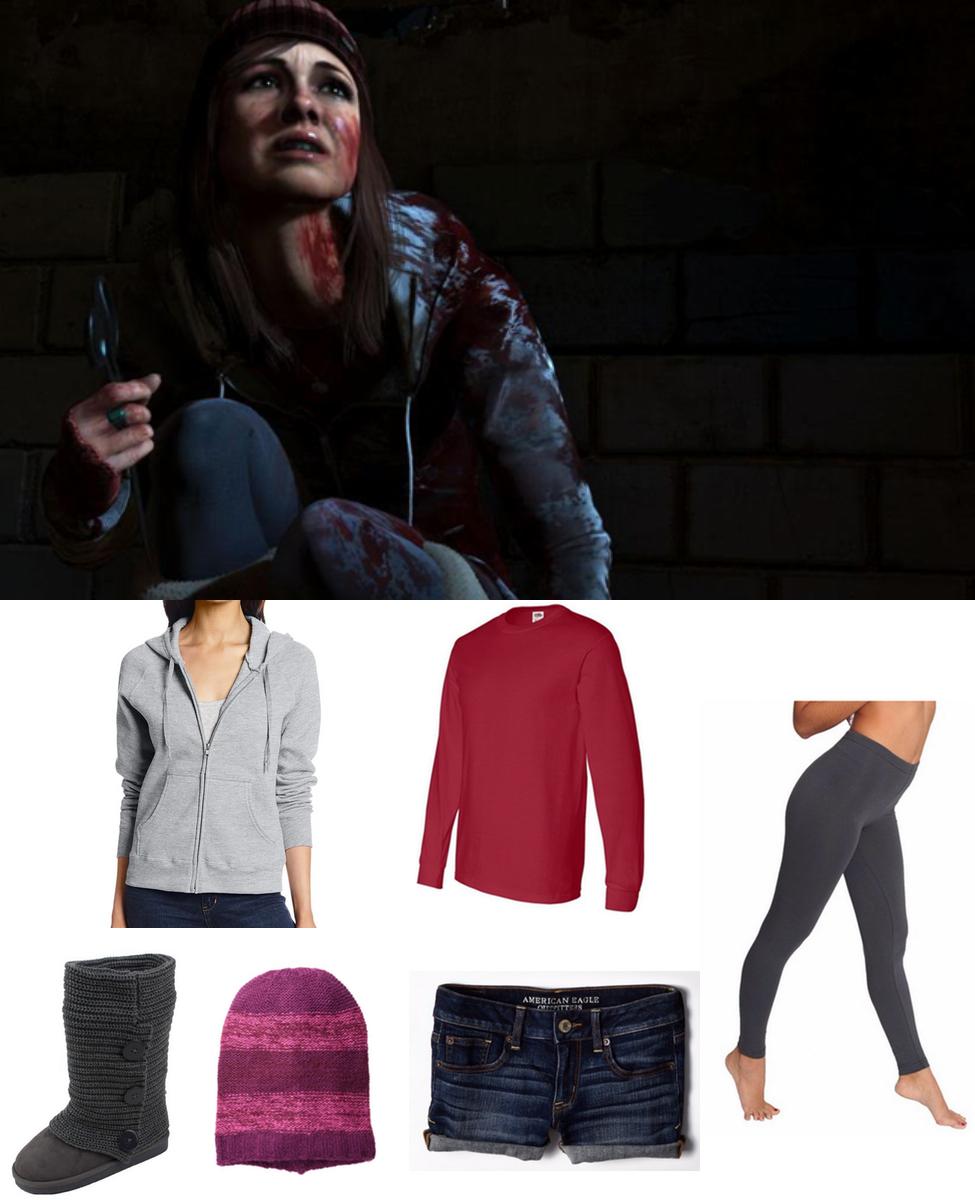The image is divided into two distinct sections, creating the impression of unrelated content. The top half features a dark and intense scene with a woman in her 20s. She has a fearful expression on her face, crouches under duress, and holds a gun in her left hand. Her leather jacket and clothing, consisting of black leggings and a black shirt, all bear splatters of blood, most prominently on the right side of her face and coat. She stands against a dark brick wall that enhances the grim atmosphere.

In contrast, the bottom half of the image has a white background and displays various pieces of clothing. This section includes a partially cut-off image of a woman in a gray zip-up hoodie and another woman in gray leggings. Surrounding these are images of different garments: a red sweater, three-button gray boots, a pink and purple winter hat, cutoff jean shorts, and other items resembling those worn by the woman in the top image. Despite their separate presentations, the clothing items in the bottom half seemingly match the attire of the distressed woman in the top half, implying a possible connection or thematic link between the two sections.